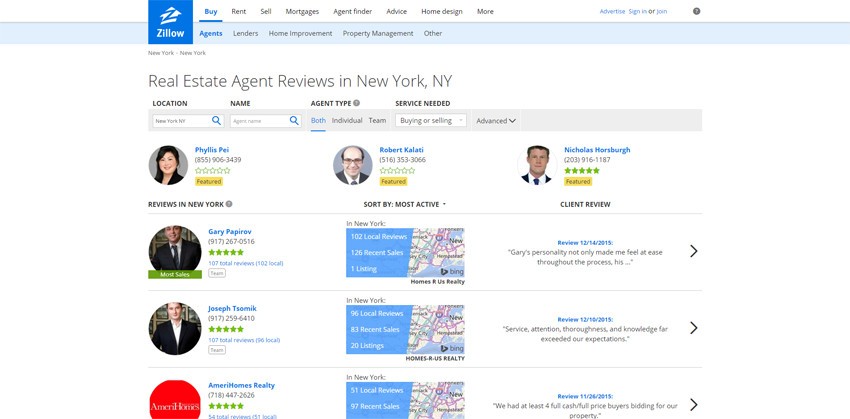This image is a detailed screenshot of the Zillow website, specifically focusing on real estate agents in New York City. Zillow, a real estate marketplace, offers resources for buying, renting, selling homes, and finding realtors. The focal point of the image features prominent gray text stating "Real Estate Agent Reviews in New York, New York."

Displayed are profiles of six realtors, each within a small box that provides the realtor's name, phone number, and links to their reviews. Accompanying each profile is a professional headshot, offering a visual introduction to the agents. 

The top of the image showcases a horizontal navigation bar with options like Buy, Rent, Sell, and Mortgages—the "Buy" section is highlighted with blue text and an underline, indicating it is the active section. Below this is another menu bar with links such as Agents, Lenders, and Home Improvement, with "Agents" highlighted in blue, pointing to the current subsection being viewed.

The screenshot captures the essence of the Zillow website's layout and functionality, clearly guiding users to explore real estate agents in New York City with ease.